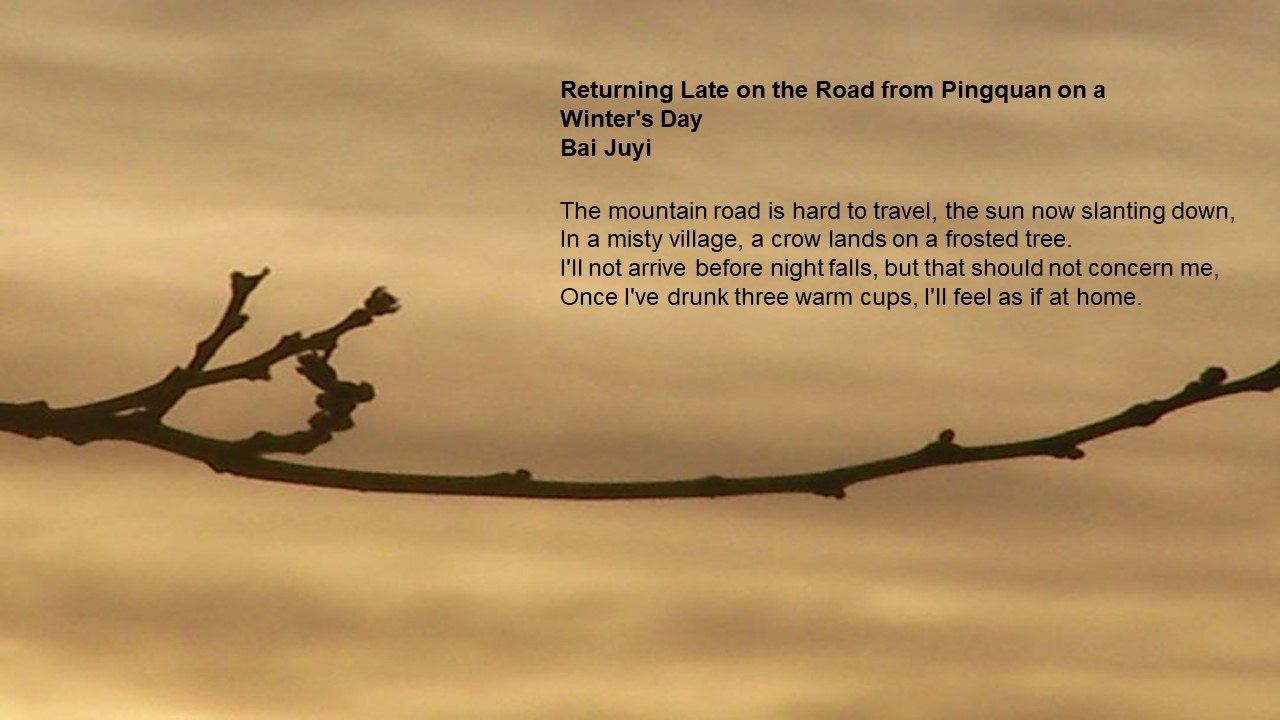The image portrays a slender, bare twig adorned with budding shoots, stretching horizontally across an out-of-focus amber and light brown sky, reminiscent of a sunset or dawn. The backdrop has a soft, sandy, almost misty appearance, enhancing the twig's silhouette effect as though taken at dusk. Scattered along the twig are a few short branches, gradually emerging against the blurred background.

In the top right corner of the image, there is black text that reads: 

"Returning late on the road from Pinguan on a winter's day, by Bì Jūyì. The mountain road is hard to travel. The sun now slanting down in a misty village. A crow lands on a frosted tree. I'll not arrive before night falls, but that should not concern me. Once I've drunk three warm cups, I'll feel as if at home."

The overall composition, with its tranquil and reflective tone, makes for a calming and meditative visual, suitable for a serene space.